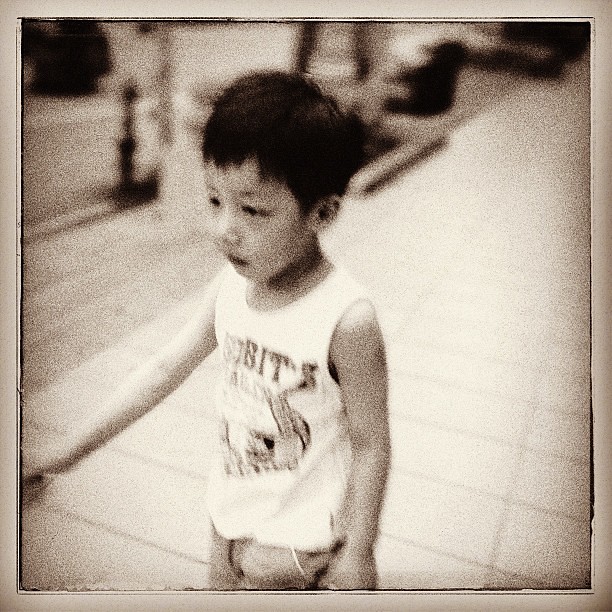In this grainy, sepia-toned Polaroid image with a matte white border, a young Asian boy, possibly around eight to ten years old, stands in the foreground as the main focus. The black-and-white image is heavily blurred, particularly in the background, which comprises what appears to be white sidewalk or cement tiling. The boy has short black hair and dark eyes, and he is wearing a white tank top that features an indecipherable graphic, possibly containing some lettering and cartoon figures. His bottoms are gray, though it's hard to discern whether they are shorts or pants. His right arm is extended out to the side, while his left hand remains close to his body as he looks off to the left. The left side of the image hints at a potential roadway or edging and perhaps a tree, though it’s obscured by the blurriness.